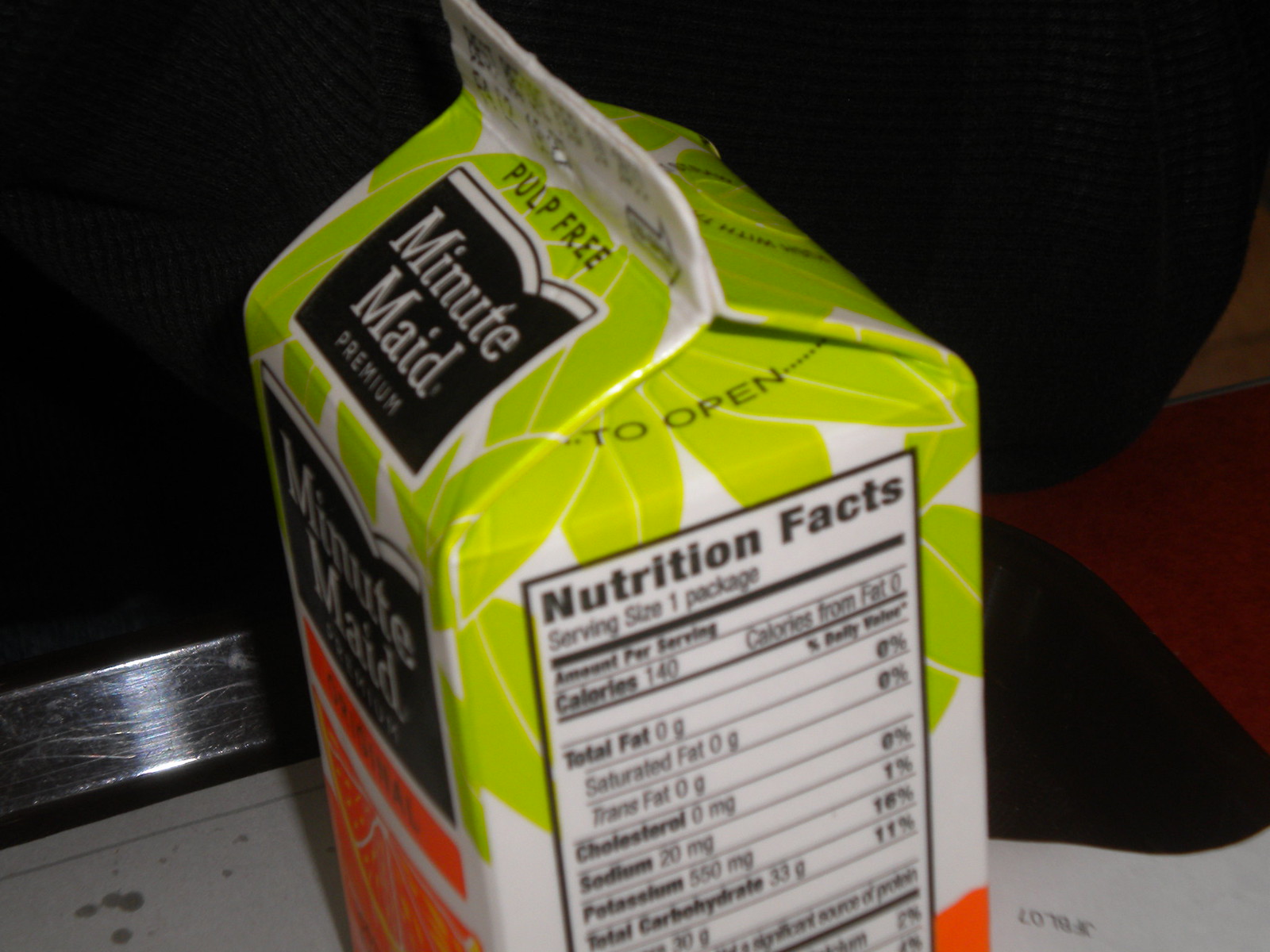This detailed photograph captures a close-up view of an unopened carton of Minute Maid Premium Pulp Free Orange Juice. The image is taken from a top-down angle, slightly to the right, showcasing the nutrition facts panel and part of the sides of the carton. The carton itself features a white background adorned with green leaves at the top and an orange section at the bottom. Printed on the front, within a black square, are the words "Minute Maid Premium" in white letters, accompanied by a picture of a half-sliced orange, suggesting the carton contains orange juice. Additionally, the carton displays a folded top with instructions on how to open it, as well as detailed nutrition information: one serving per package, 140 calories, 0g fat, 0g saturated fat, 0g trans fat, 0mg cholesterol, 20mg sodium, 550mg potassium, and 33g carbohydrates. In the background, there is a metal bar, some black object to the right, and a red material that could be carpet or fabric, all situated on a table or surface.